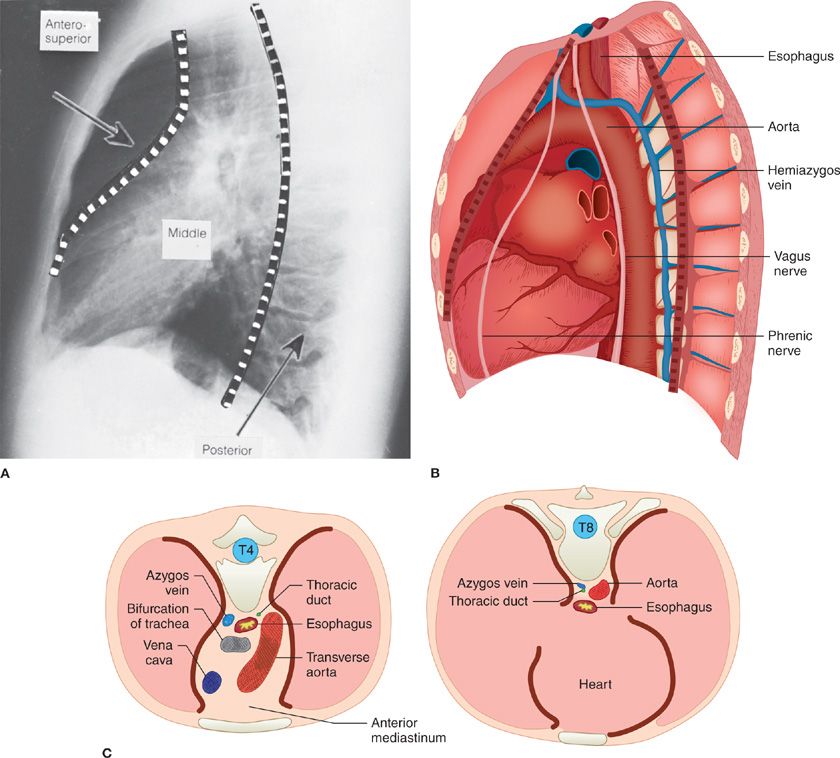This scientific informational graphic provides detailed visualizations of the esophagus and surrounding anatomical features within the chest cavity. The graphic includes four distinct images. Image A, situated at the top left, is a black and white x-ray of the chest cavity taken from a lateral view, highlighting the spine, lungs, and different sections of the esophagus within the anterior, middle, and posterior mediastinum. Image B, located at the top right, is a labeled anatomical diagram that mirrors the x-ray and illustrates the esophagus, aorta, various veins, and nerves such as the azygous vein, vagus nerve, and phrenic nerve. Image C, at the bottom, is composed of two cross-sectional views presented side by side. These circular slices offer a transverse perspective, showing distinct anatomical features including the vertebrae, lungs, aorta, bifurcation of the trachea, vena cava, thoracic duct, and esophagus from different orientations. The cross-sectional images provide a comprehensive view of the thoracic structures relevant to the esophagus’ anatomical context.